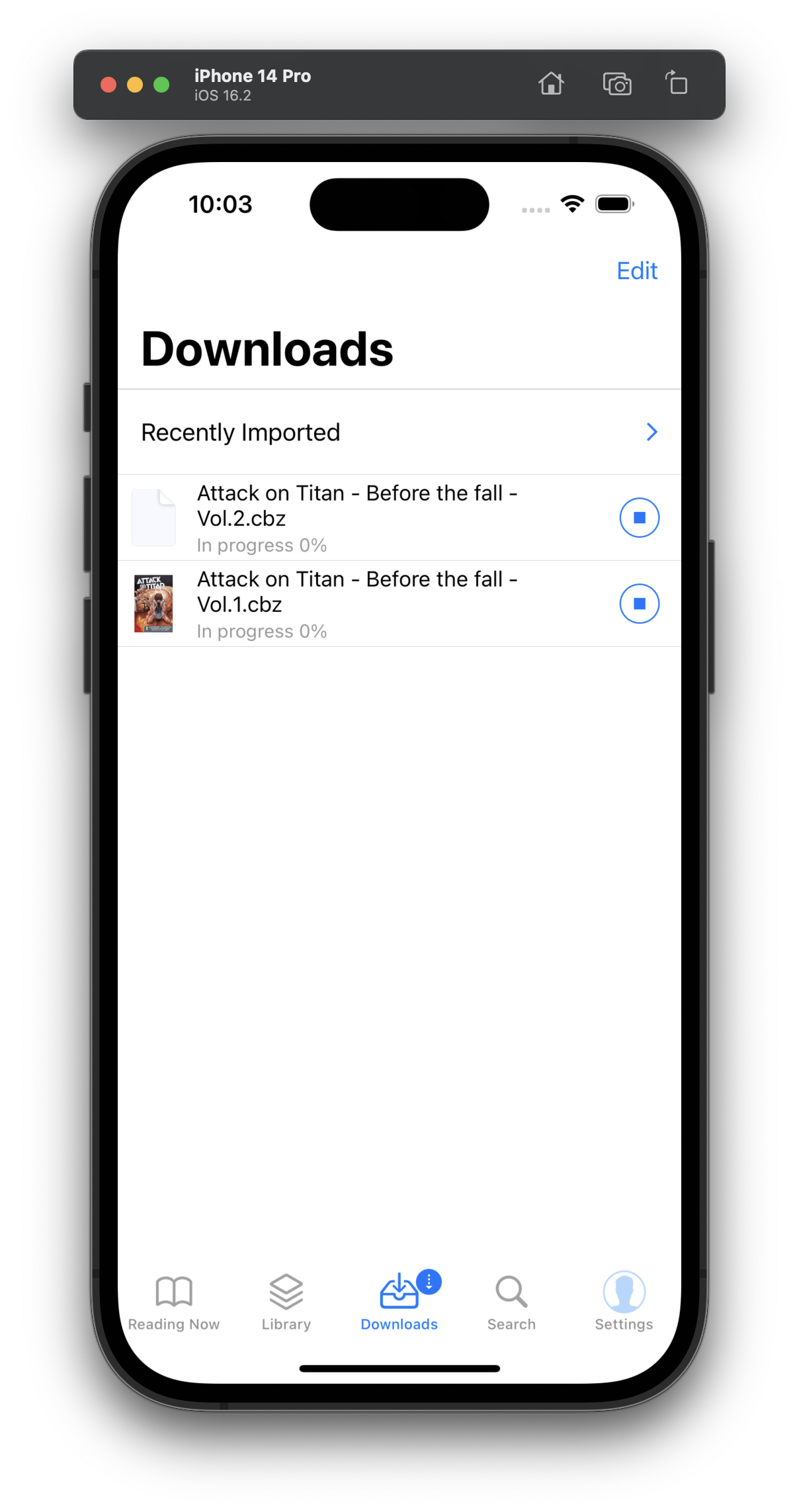The image displays the screen of an iPhone 14 Pro, which is using the iOS 16.2 operating system. At the top of the screen, there is a gray rounded rectangle filled in completely. Inside this rectangle, positioned near the middle left, are three dots—red, yellow, and green, arranged in that order. Above these dots is the text "iPhone 14 Pro" in white, while "iOS 16.2" appears in gray text underneath.

In the top right corner of this gray rectangle, there is a small square with an upward arrow located in the top left corner of this square. Next to it are icons for a camera and a house, moving from right to left. 

The main part of the phone screen shows the time "10:03" in black text at the top center. To the top right of the time, there are icons for Wi-Fi and battery status. Directly beneath the battery icon, the word "Edit" is displayed in blue text.

Below the time, there is a large black text that reads "Downloads," accompanied by a thin gray horizontal bar underneath it. Further down, the text "Recently Imported" appears, with a blue arrow pointing to the right located on the far right of this label.

Under "Recently Imported," there are two download items listed. The first download has an icon of a piece of paper with a bent top-right corner, indicating a document, and is labeled "Attack on Titan: Before the Fall, Volume 2." Directly below it, another item labeled "Attack on Titan: Before the Fall, Volume 1" is shown. To the right of each download item, there is a blue stop button.